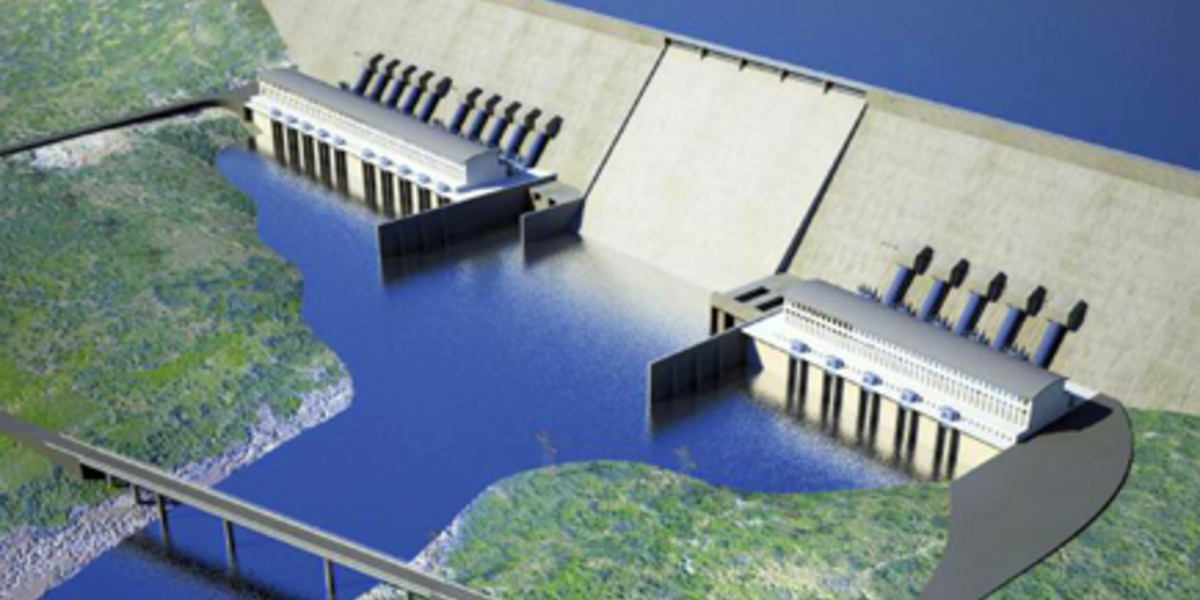The image depicts a detailed, somewhat stylistic rendering of a dam, possibly from a video game or a painting. In the upper right-hand corner and across the background, there is a large body of blue water, suggesting a reservoir. The central structure is a large, white, brick-like dam stretching across the water, with significant cement infrastructure and locks on both sides. Attached to the dam are buildings with blue, smokestack-like structures protruding; there are five on one side and ten on the other. The dam is outlined in black, with a tan band that features intricate lines possibly indicating fencing. The surrounding landscape includes green land on both sides of the water. Additionally, at the very bottom of the picture, a bridge spans the gap between the dam's lake and the adjacent land. The setting combines elements of water and terrestrial scenery, providing both structural and environmental detail.